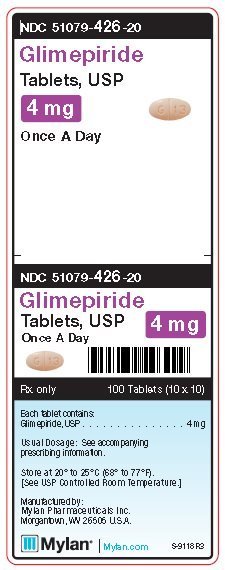The image depicts a medication box that is divided into multiple labeled sections. The top section bears the information "NDC 51079-426-20" and states "Glimepiride Tablets, USP, 4 mg, once a day." There is an accompanying image of a small pill. Below this section is another label with the same NDC number, "51079-426-20," and the text "Glimepiride Tablets, USP, once a day, 4 mg." To the right of this text, a barcode is displayed alongside the same pill image from the top section. Additional details on the box include: "Rx only, 100 tablets, 10x10," and further information clarifying that "Each tablet contains Glimepiride USP, 4 mg." The usual dosage instructions prompt users to refer to the accompanying prescription information. Storage instructions indicate to keep the medication at 20°C to 25°C (68°F to 77°F) in a USP-controlled room temperature environment. The box specifies that it is manufactured by Mylan Pharmaceuticals Inc., located in Morgantown, West Virginia, USA, with the code "6505." It also references Mylan's website, "Mylan.com," and additional identifying marks, "S9118R3."